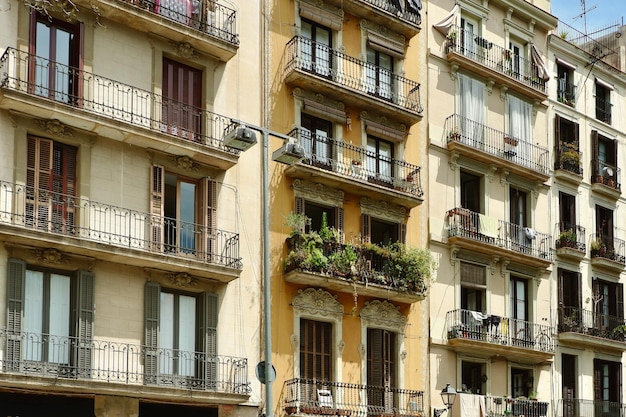This image depicts an apartment complex that appears to be situated outside the United States, potentially in a European or Central American setting. The complex is at least five stories tall, possibly taller, given that the bottom levels are cut off in the photo. The buildings feature various shades of off-white, beige, tan, orange, and a yellowy-gold color, creating a rich, warm palette. Each apartment unit has a wrought iron balcony that is a dark brown color. These balconies have two doors, either glass doors trimmed with wood or plain brown wooden doors. Some balconies are split into two separate sections, though most are single, spacious balconies encompassing two doors. The middle section of the complex stands out with a balcony lushly decorated with plants, while other balconies have modest displays of plants, bicycles, and chairs. Many balconies, particularly on the far left and right, appear sparsely decorated. The buildings are characterized by numerous windows, some of which are open and some closed, adding to the dynamic appearance of this vibrant, urban apartment complex.